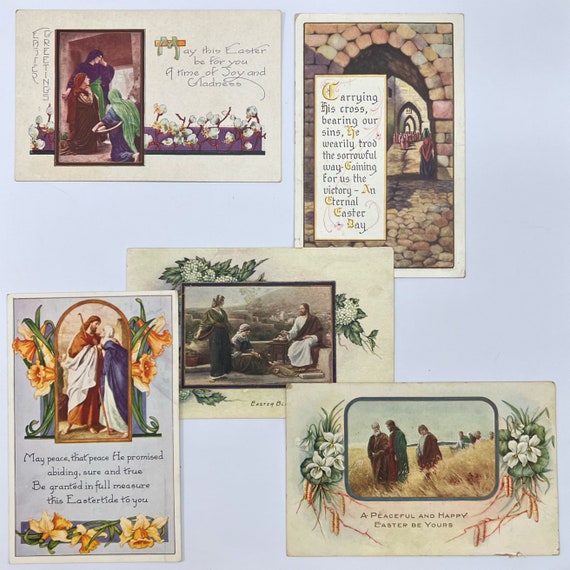The image is a square collage of what appear to be Easter and possibly Christmas greeting cards, all displayed on a large grey background, likely resembling a wall display. Each card features traditional, almost medieval or biblical illustrations. People depicted in the scenes are wearing robes, tunics, and head coverings, evoking a historical or scriptural aesthetic. Prominent figures such as Jesus and Mary appear in various scenes – for example, Jesus walking with a staff and Jesus with Mary. The cards are written in multiple languages, with black text that includes messages such as "Carrying the Cross," "Bearing our Sins," "A Peaceful and Happy Easter Be Yours," and other greetings wishing peace and happiness. Many of the cards also incorporate floral motifs. The color scheme for the images includes grey, white, green, and purple in the outfits, rendering a faithful yet varied presentation of each card.